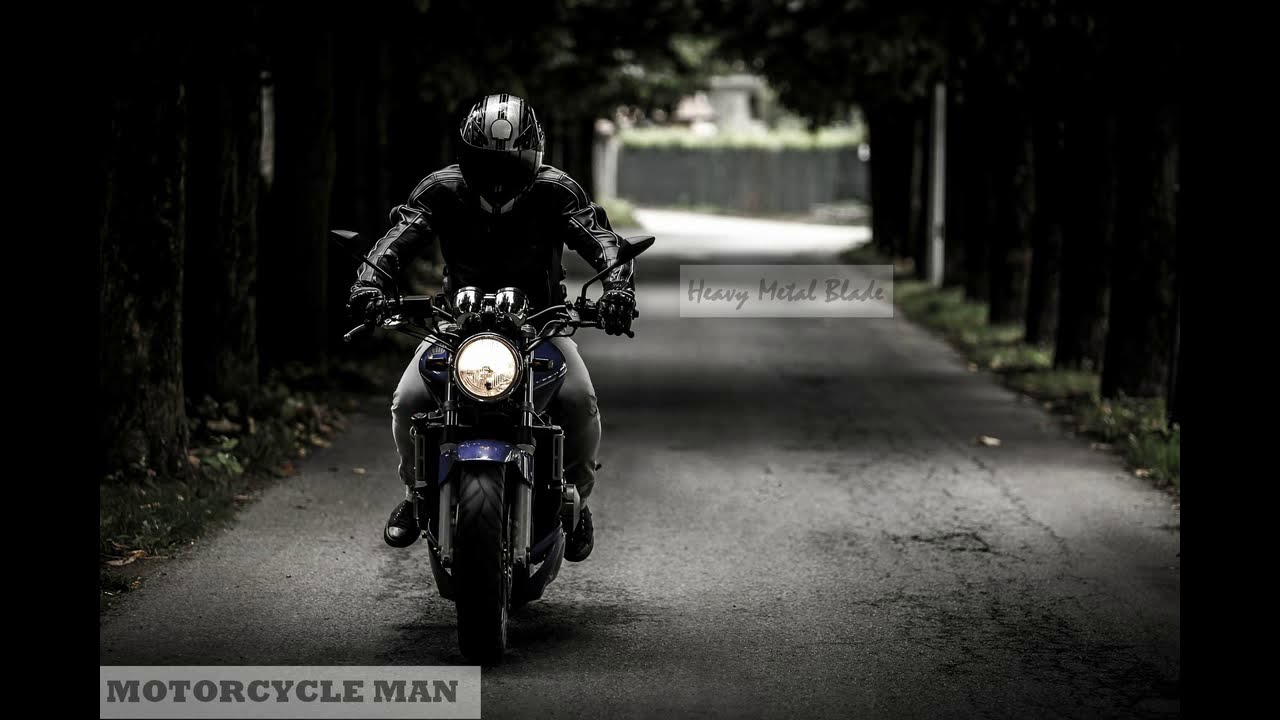In this atmospheric outdoor scene, a solitary man rides a blue motorcycle down a gravel road flanked by tall, shadowy tree trunks, with the lush foliage forming an arch of branches laden with leaves towards the back of the image. He is dressed in an ensemble of black, including a sleek black helmet with a silver stripe obscuring his face, a black leather jacket, black pants, and black gloves. You notice that the road begins at the bottom of the image and gradually fades into the distance towards the middle-top. On the lower left, a gray box with the bold, capitalized text "Motorcycle Man" stands out, while the center of the image prominently features the cursive inscription "Heavy Metal Blade" in another gray box. Fallen leaves speckle the grassy verge at the bottom of the scene, adding a touch of autumnal scenery, and in the far background, beyond the trees and the road, you can glimpse a building and a fence.